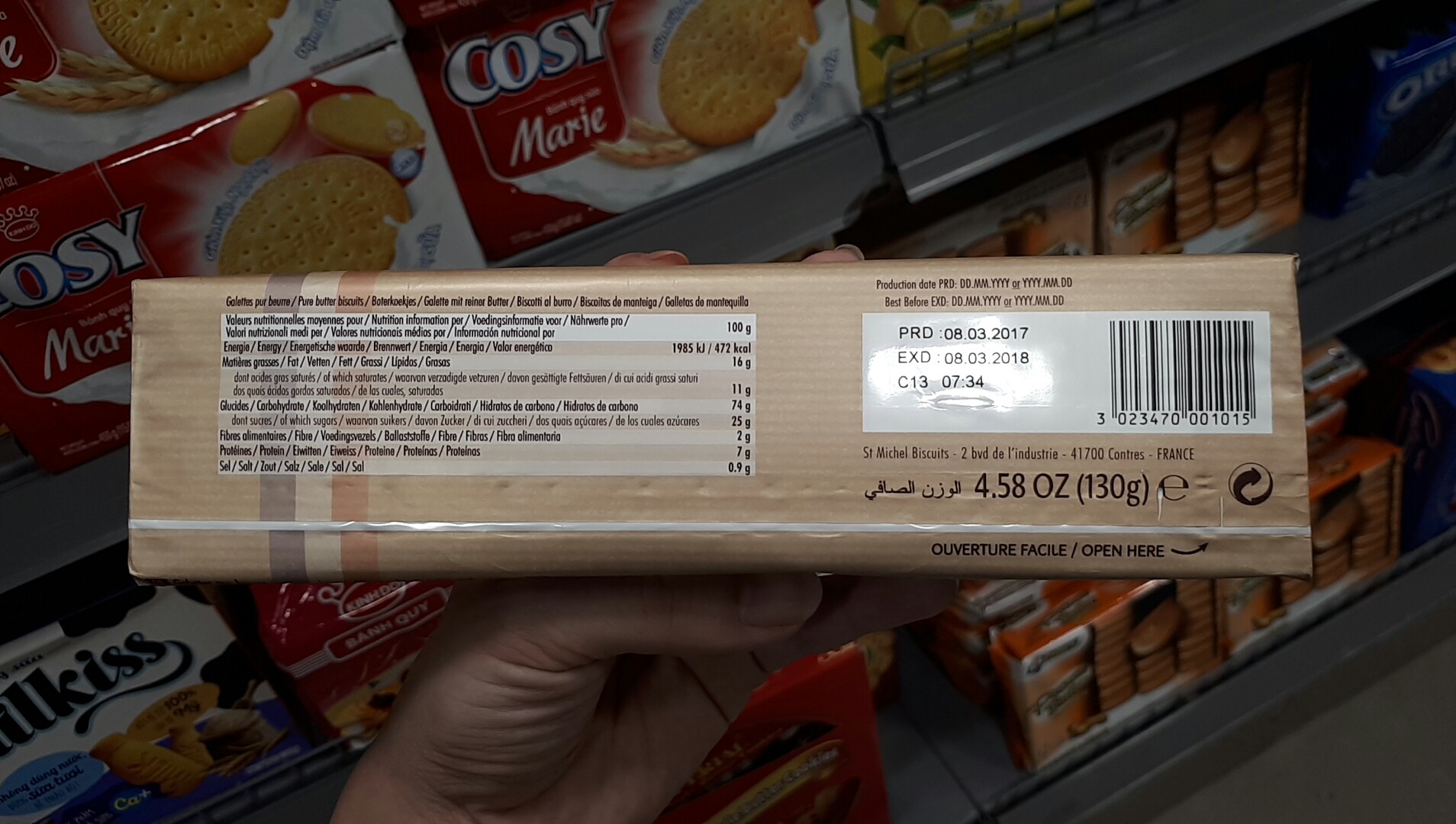In this dimly lit interior shot taken at a slight angle, a left hand emerges from the lower left of the frame, holding a long, narrow, rectangular tan package horizontally. The package displays a large black and white text box on the left side listing nutritional information, including "472 kcals" and "16 grams fat," albeit in a font too small to be easily read. Adjacent to this, the label features a white rectangle containing the production and expiration dates, along with a barcode and other small text details such as "4.58 ounces (130 grams)." There is a slight glare on the package, possibly from store lighting or a camera flash. The background reveals a grocery store setting with shelves filled with various items, including what appear to be Cozy Crackers, a brand associated with "St. Michael Biscuits" from France, along with other recognizable products like cheese and cracker sandwiches, and a pack of Oreos. The label also mentions the word "Marie" and depicts a round cracker.